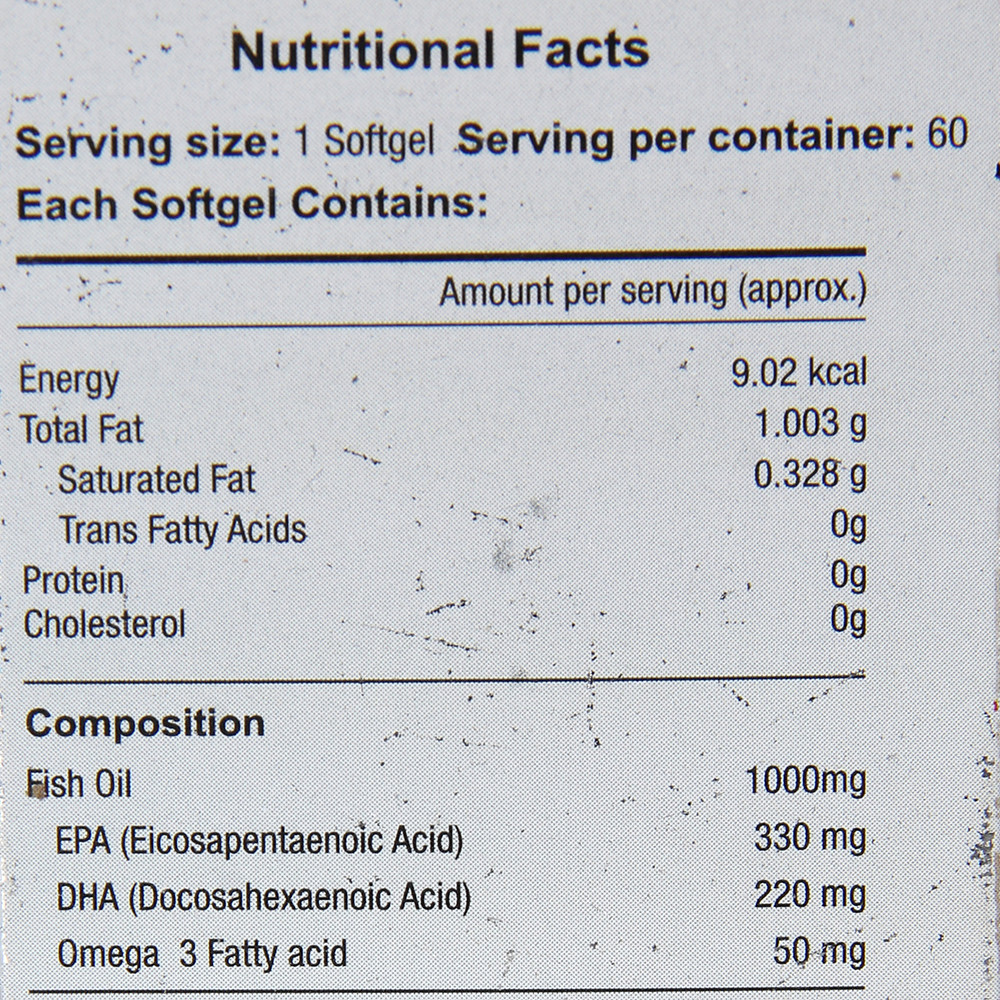The image depicts a slightly scuffed nutritional facts label on a white background. At the top, bold black letters indicate "Nutritional Facts." The label details that each serving size is one soft gel, and there are 60 servings per container. Each soft gel provides 9.02 kilocalories of energy, 1.003 grams of total fat, including 0.328 grams of saturated fat, 0 grams of trans fatty acids, 0 grams of protein, and 0 grams of cholesterol. The composition section lists that each soft gel contains 1,000 milligrams of fish oil, which includes 330 milligrams of EPA (Eicosapentaenoic Acid), 220 milligrams of DHA (Docosahexaenoic Acid), and 50 milligrams of other omega-3 fatty acids.